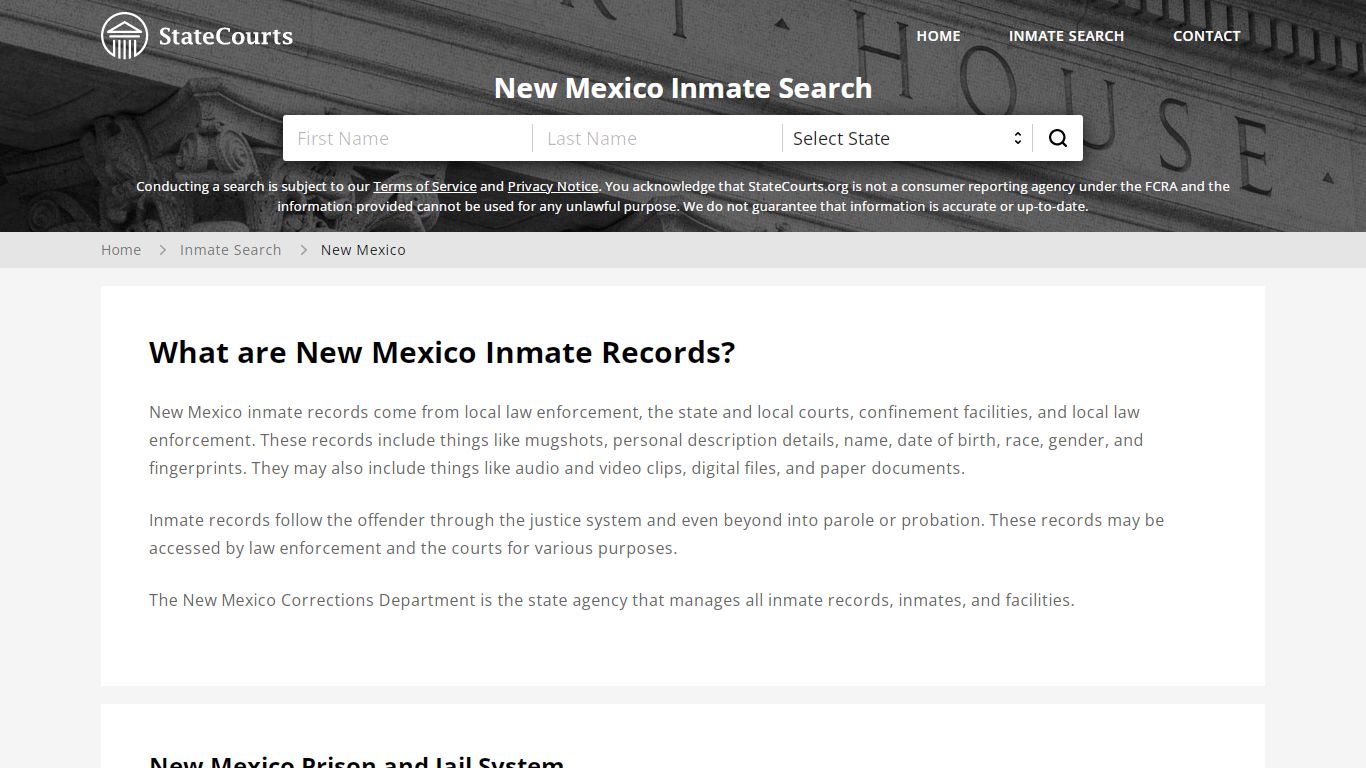The image depicts a minimalist room characterized by its simplicity and straightforwardness. Dominated by a neutral color palette, the space lacks any vibrant or standout elements, reinforcing its utilitarian design. The layout is clear and unambiguous, offering no extraneous features or potential distractions. This room prioritizes functionality, providing only the essential information and elements needed, making it nearly impossible to get lost or confused. The straightforward design is appreciated by those who prefer clarity and directness, ensuring that all necessary information is immediately accessible and unadorned.